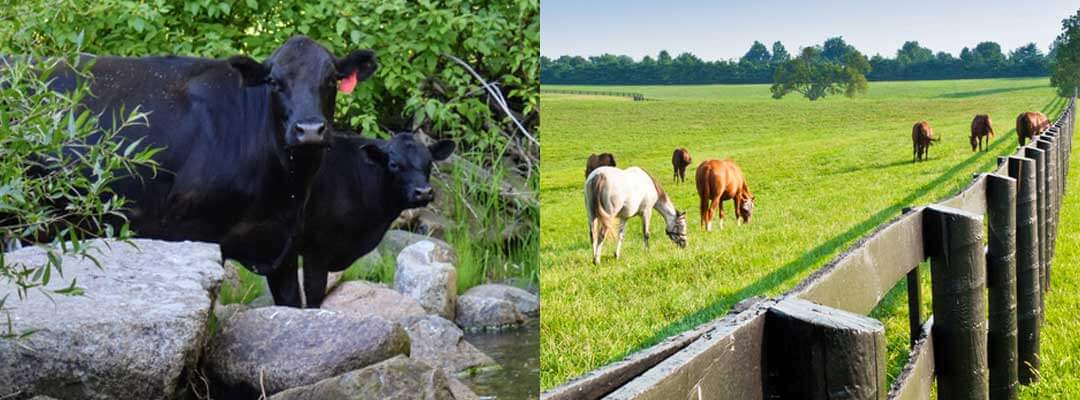The image is a split-panel photograph taken during the daytime. The left panel features two large black bulls or cows standing amidst a landscape of gray boulders and surrounding greenery, including shrubs and trees. The animals face to the right, standing chest-high behind the rocks. There's also a hint of water visible around the cows.

The right panel shows a vast grass field with a wooden fence extending from the lower center to the upper right corner. Around seven horses are grazing in the field, predominantly brown with one white horse bearing a brown tail. The background is dotted with trees, including one prominent tree in the center of the field and another in the upper right corner. Both panels capture the serene outdoor environment under a blue sky, with the overall setting framed by lush green grass and dense trees in the distance.